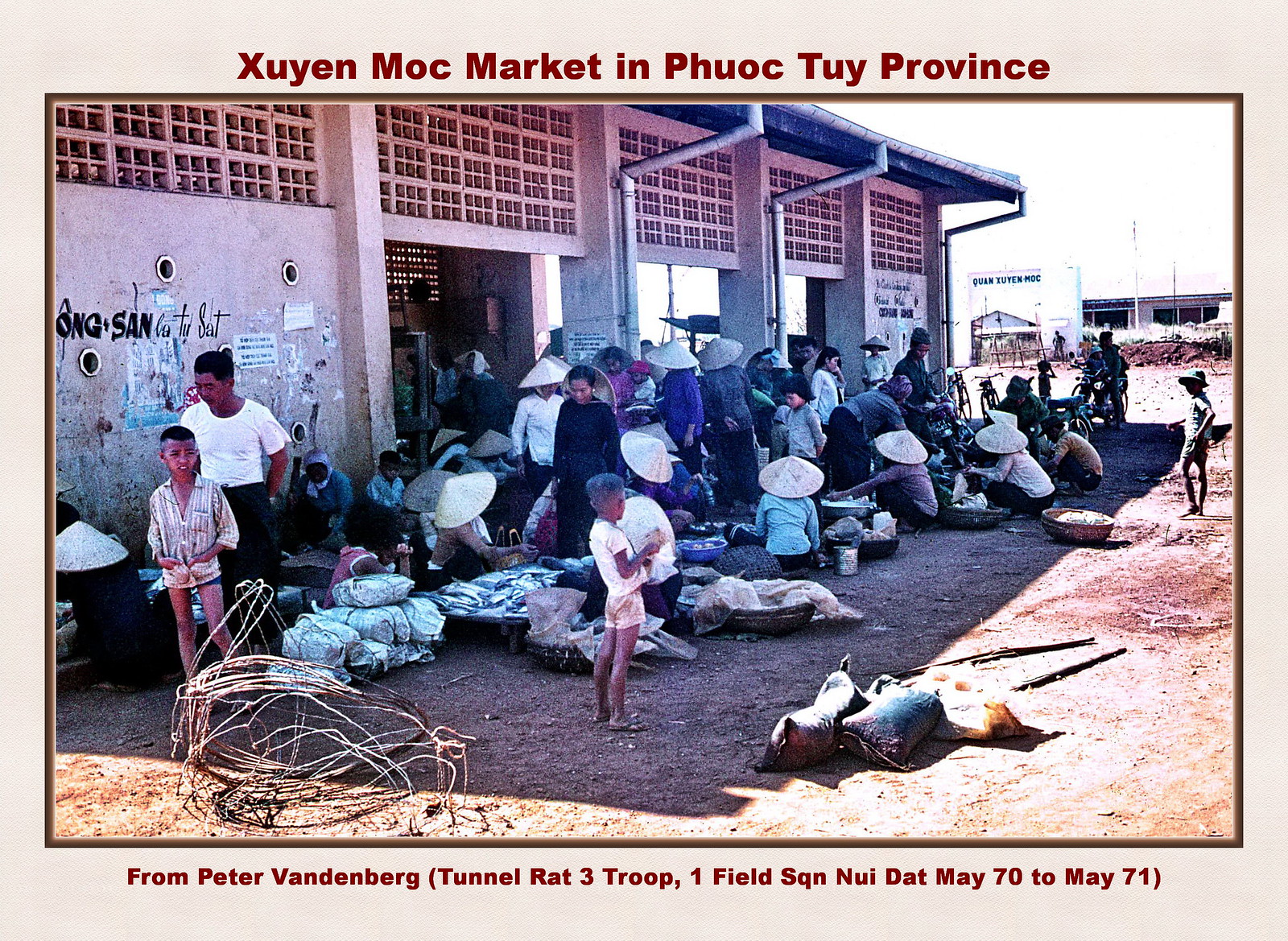The detailed photograph captures a bustling scene at the Zuyen Moc Market in Phuoc Thuy Province, as indicated by the red text above the image. This market area is framed by a gold outline and shows a dirt-ground setting with various vendors and patrons. The vendors, some wearing traditional conical rice paddy hats, have their goods displayed on the ground, primarily in woven baskets and bags, which appear to contain food items and other merchandise. The scene is chaotic, with items strewn about and the market seemingly lacking organization. Vendors are either seated on the ground or standing by their goods, engaging with potential buyers. The backdrop includes a gray-walled building with minimal doors, photographed from a diagonal angle. Additional text on the right side of the image reads "Kwan Zuyen Nok" in black font. Below the image, in red text, it states, "from Peter Vanderberg (Tunnel Rat 3 Troop, one field, SQN, Nui Dat May 70 to May 71)." The photograph offers a vivid glimpse into the day-to-day activities and conditions of a market in this region of Asia.